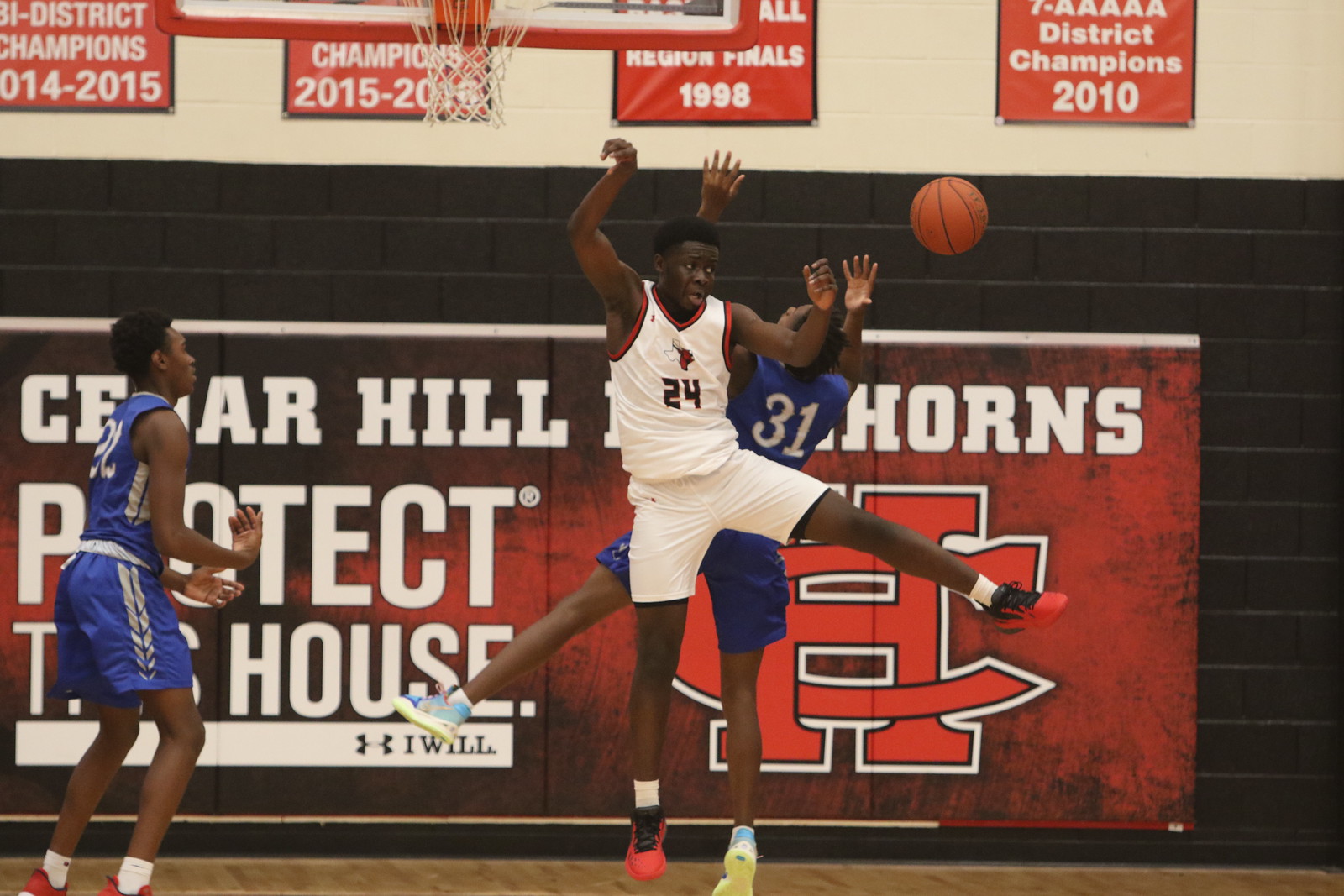In this vibrant indoor photograph of a high school basketball game, we witness an intense moment of action. The scene is set on the polished wooden floor of a gymnasium, framed by a dark brick wall adorned with banners celebrating Cedar Hill's basketball achievements, including District Champions 2010, Regional Finals 1998, Champions 2015, and District Champions 2014-2015. Prominently displayed are the words "Cedar Hill, protect this house," along with the Cedar Hills emblem.

At the heart of the image are three dynamic players. In the foreground, a player in a white uniform with red trim, numbered 24, leaps into the air, arms stretched skyward and eyes focused intently on the orange basketball hanging midair. His red and black sneakers contrast sharply with his white attire. Close behind him, another player in a blue uniform marked with the number 31 and white digits, also jumps with his hands reaching up, wearing blue and yellow shoes. His back is turned towards the player in white, creating a dramatic back-to-back scene. To their left, another athlete in a blue uniform, sporting red shoes, stands on the ground, his attention fixed on his airborne teammates. The energy and athleticism of the game are palpable, capturing the spirit of high school basketball at its finest.